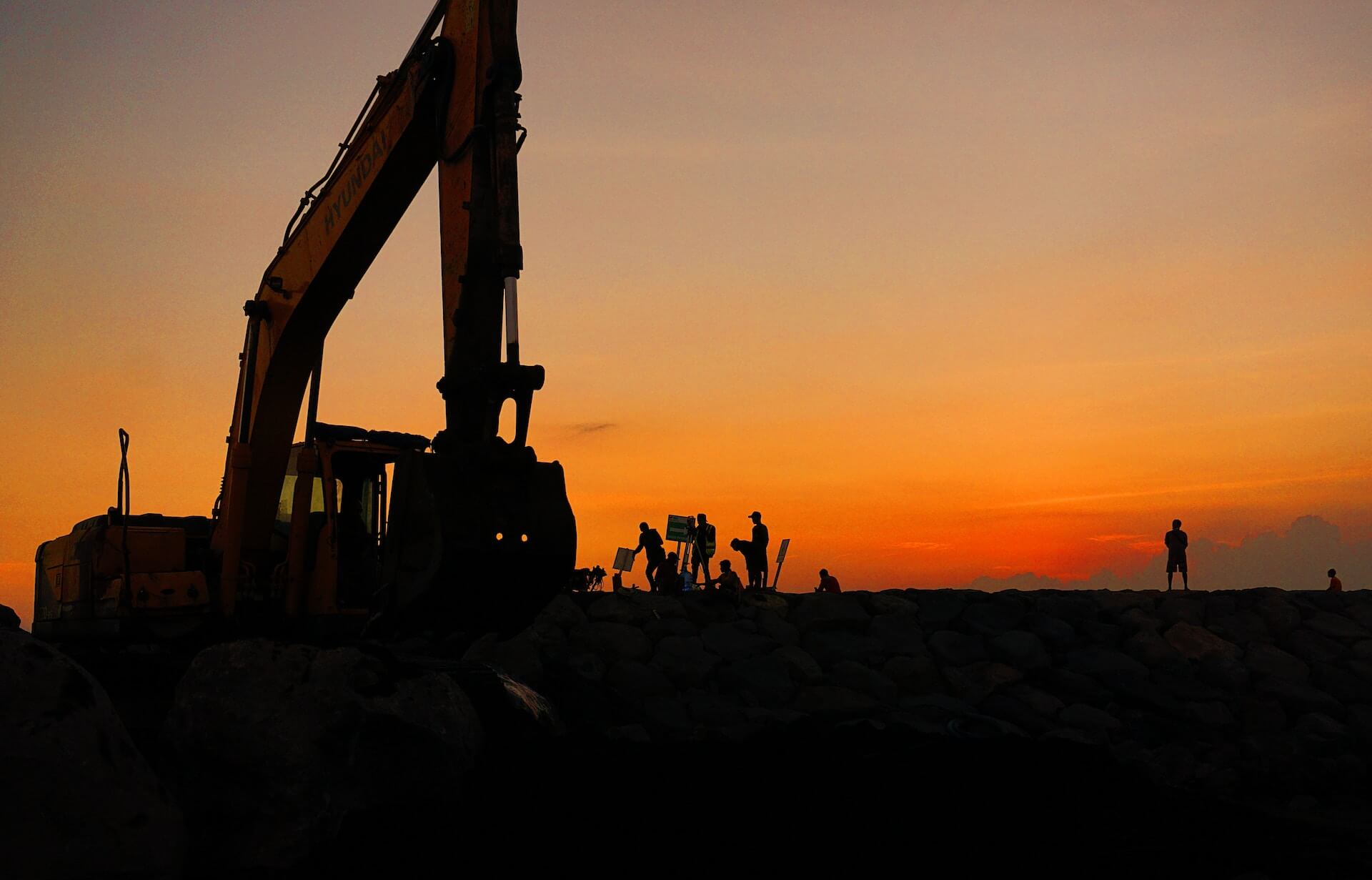In the dim light of either sunrise or sunset, this color photograph captures a tense scene dominated by a large, yellow excavator positioned on the left. The machine's cab is clearly visible, along with its intricate hydraulic arm extending upward before bending at a 90-degree angle to support a hefty bucket. Across the rocky, boulder-strewn landscape that occupies the lower portion of the image, silhouettes of around a dozen people appear, half sitting and half standing, engaged in what seems to be a protest. Some hold signs, adding to the palpable sense of opposition against the ongoing construction suggested by the excavator. The background transitions from a red horizon to a mellow yellow, climaxing in a gray sky above, casting a beautiful yet dramatic orange hue over the scene. While the main action centers on the left, a few individuals are scattered further right; one person stands, looking at the horizon, while another peeks just above the rocks, observing the protest with their back turned to the camera.